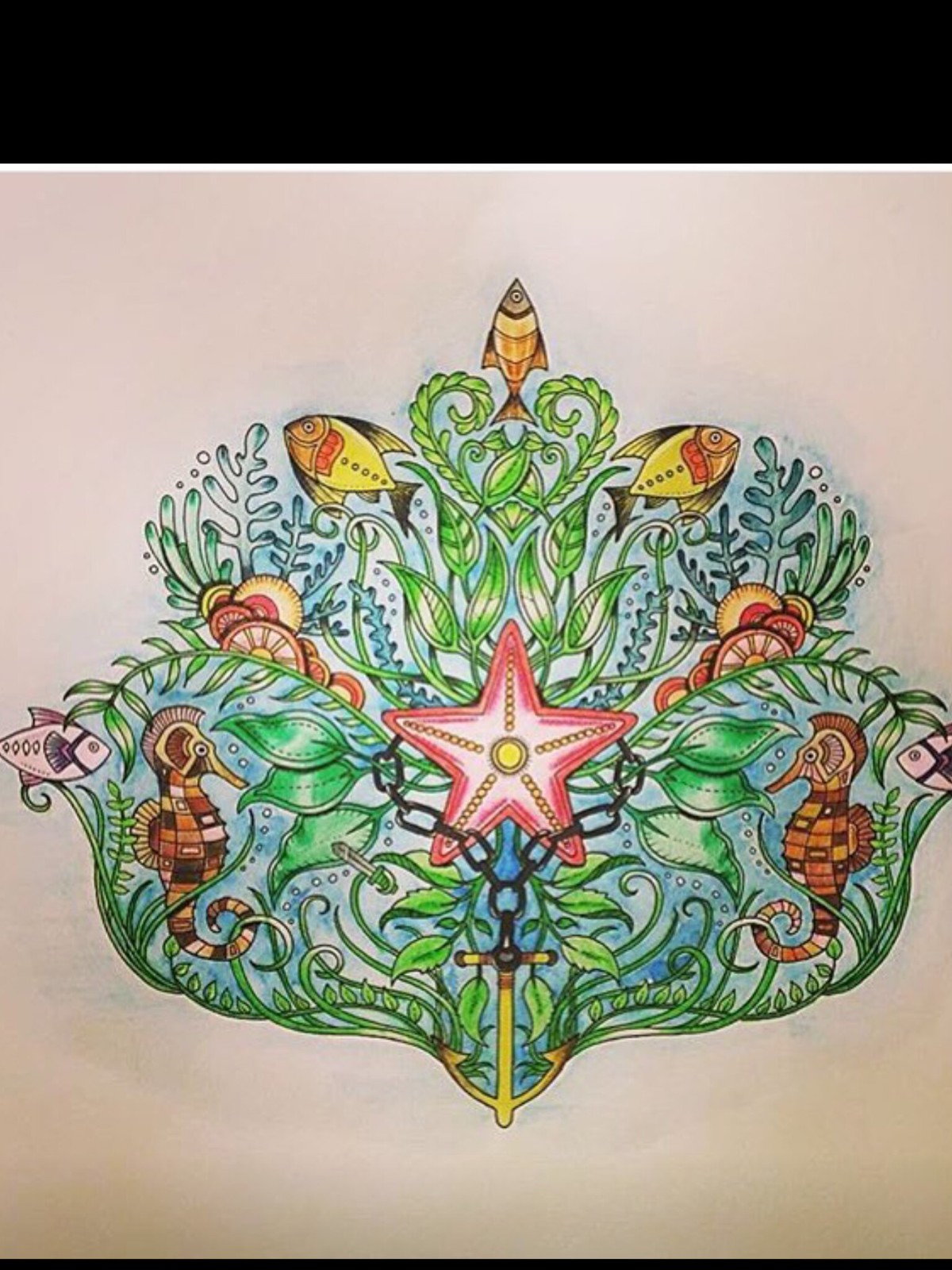This intricate piece of artwork, set on a white canvas with hints of a cream undertone and framed against a narrow black background, features a vivid underwater theme. Central to the composition is a prominent pink starfish, surrounded by a black chain with a golden cross pendant. Two brown seahorses, each facing inward towards the starfish, flank this focal point. The aquatic scene is further enriched by five other fish: two pink fish positioned behind the seahorses, three yellow fish with one at the peak of the composition, and a varied mix of colors including brown and red. Interwoven and curling throughout are vibrant, detailed green seaweed and kelp, adding to the lush underwater tapestry. The scene is painted with an array of bright colors like green, blue, orange, yellow, and pink, contributing to a beautifully ornate and dynamic collage, reminiscent of a fleur-de-lis shape.